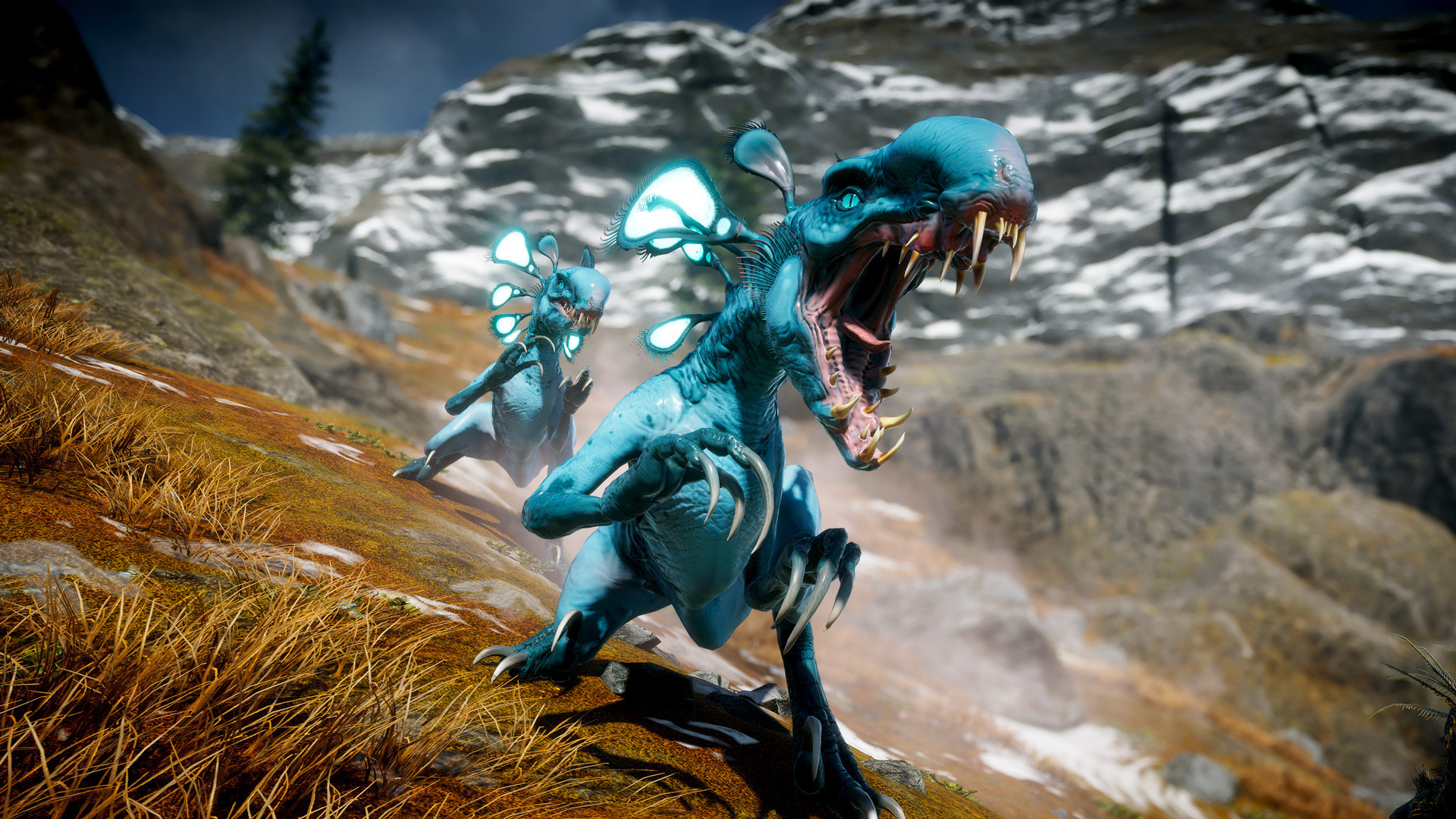The image is a captivating screenshot from the video game "Second Extinction," featuring a vividly-rendered, turquoise-blue alien-like dinosaur creature as the central focus. The monster stands prominently in the foreground, showcasing massive, razor-sharp teeth in its wide-open mouth, with its tongue partially protruding. It possesses large claws, long arms, short feet, and a head reminiscent of a dinosaur's. A second, smaller alien-dinosaur creature, nearly identical in appearance but with a closed mouth, can be seen directly behind it. The environment depicts a rugged, rocky landscape with a mountain in the background, its crevices dusted with snow. A slightly tilted pine tree adds a touch of realism to the scene. The background elements are out of focus, emphasizing the ferocious nature of the approaching creature.